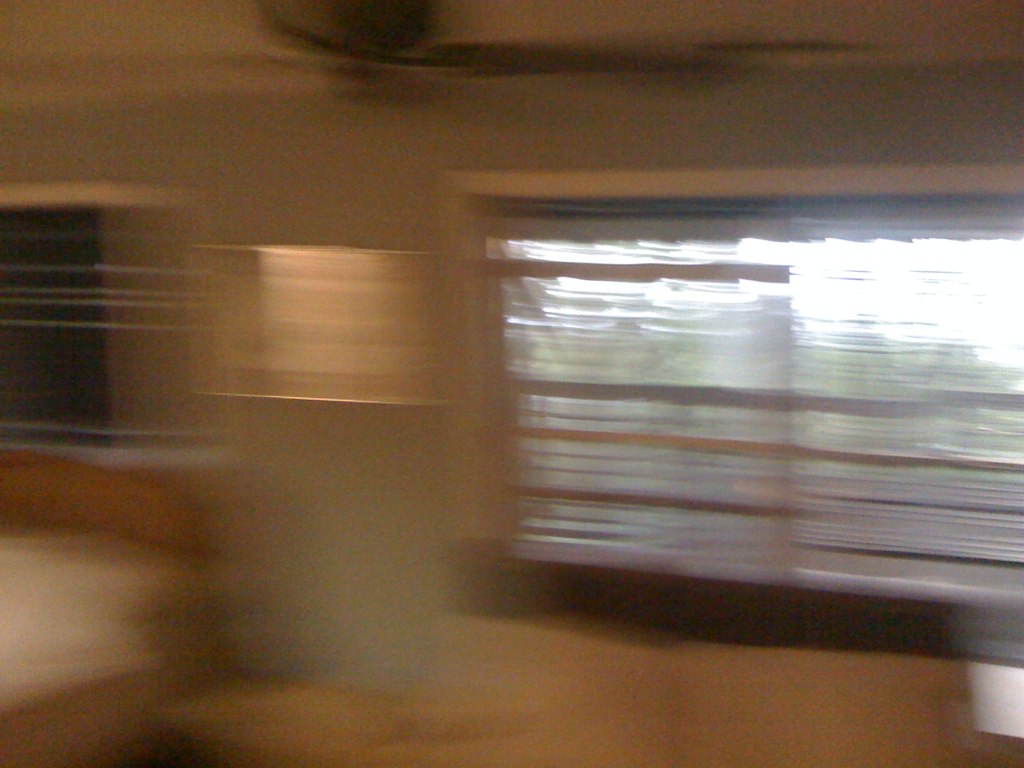The image is a highly blurred interior shot of a room, creating a fuzzy and smeared appearance throughout. Dominating the right side is a window with blinds, highlighted by a white windowsill or door frame. Above this, in the upper portion of the image, a light brown ceiling fan is faintly visible due to the image distortion. To the left of the window, a wall light appears, its size exaggerated by motion blur. The bottom left corner showcases part of a bed with a wooden frame. The lower section of the image features various indistinct objects resembling a light brown blur, including hints of a hardwood floor. The center left side potentially displays a bright area, possibly a door, while the overall color scheme suggests gray walls trimmed in white, interspersed with wooden panels and rails.